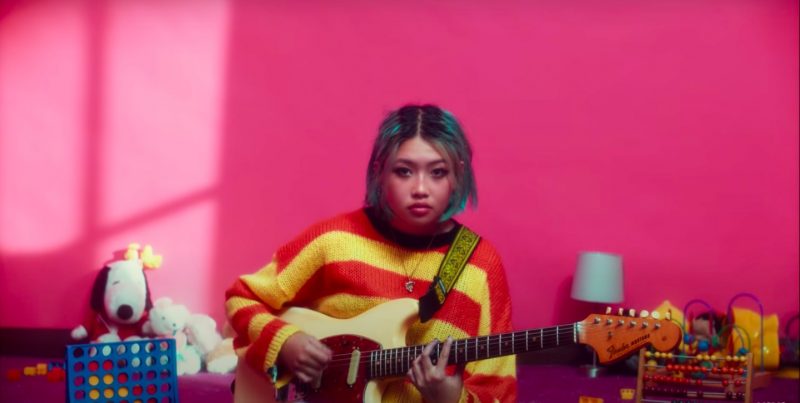The image captures a young Asian woman with a stylish bob haircut, featuring black roots that transition into a striking teal blue, just an inch and a half above her shoulders. She is wearing a bold red and yellow striped sweater, complemented by a silver necklace nestled against a black collar. A guitar strap is slung over her shoulder, and she is holding a white electric guitar, mid-strum, her gaze directed at the camera with a confident, makeup-adorned face. The vivid background of the room is painted a vibrant hot pink, creating a playful and energetic atmosphere. To her left, there is a Snoopy doll among several other stuffed animals, as well as a Connect Four game with blue, yellow, and red pieces. On her right, a small white lamp sits next to an abacus with colorful beads, surrounded by other childhood toys, including a few building blocks. The overall scene is one of colorful chaos, reflecting both a sense of youthful creativity and musical passion.